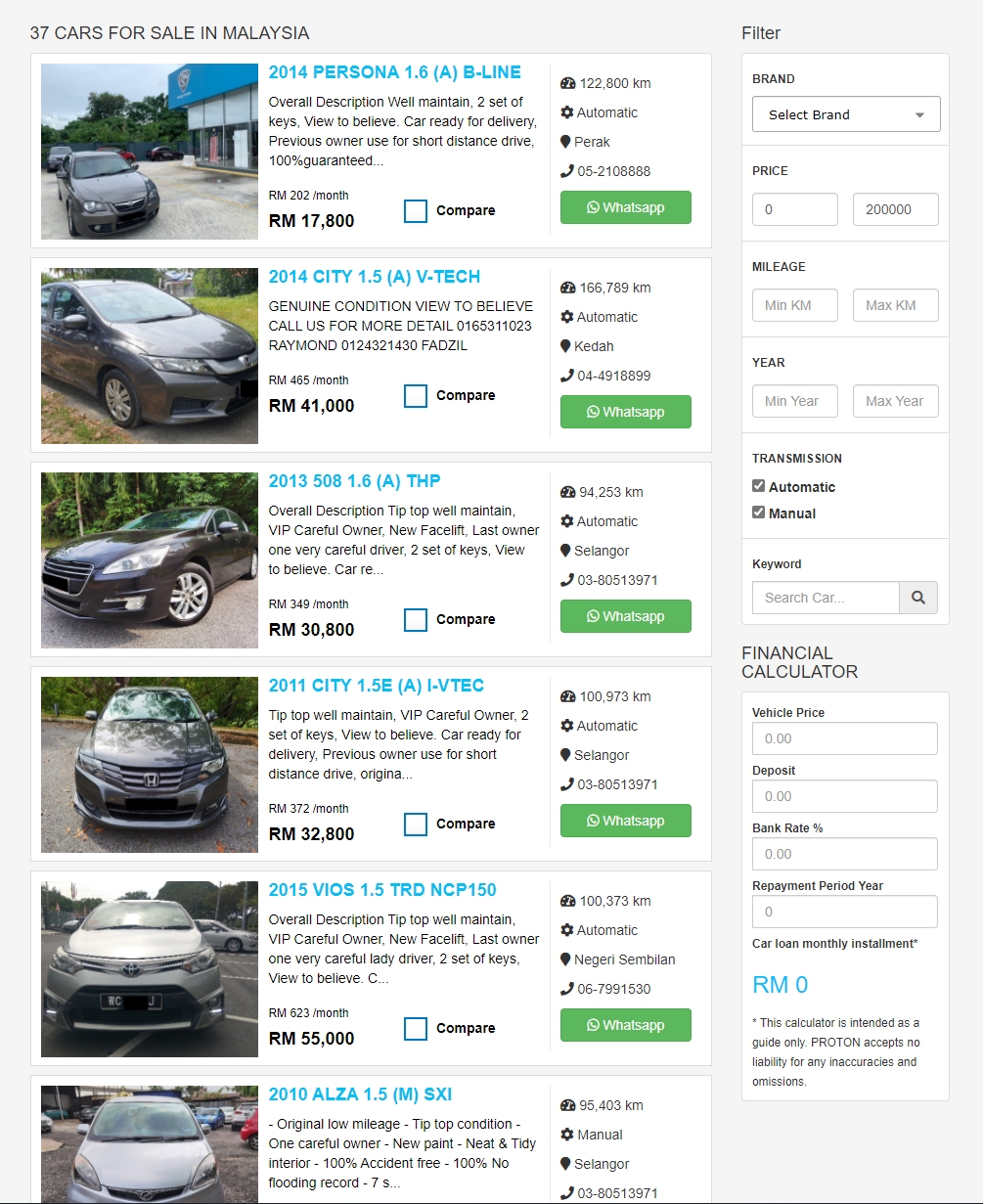The webpage is a car sales platform featuring a diverse selection of vehicles available in Malaysia. At the top left, a heading indicates "37 cars for sale in Malaysia." Beneath this, six prominently displayed car listings fill the page, each accompanied by high-resolution images predominantly showcasing various sedan models, characterized by their four doors.

Each car entry includes detailed information clearly formatted in columns. The first listing features a 2014 Persona 1.6 AB. Below the main heading, a thorough description outlines the car's condition as "well-maintained, with two sets of keys. The vehicle is ready for delivery and was previously used for short-distance drives, boasting a 100% guarantee." The price is listed as "RM 17,800." Additional details specify the car's mileage, type (automatic), along with a contact phone number and a WhatsApp number for inquiries. The subsequent five car listings maintain a similar structure, consistently providing vital information such as the car model, a brief description, price, mileage, type, and contact details.

To the right of the car listings, a user-friendly filter panel allows potential buyers to refine their search. The filter options include a drop-down menu for selecting the car brand, as well as fields to specify price range, mileage, and the year of manufacture. At the bottom of the filter section, a financial calculator aids users in planning their purchase by calculating potential payments based on the listed prices.